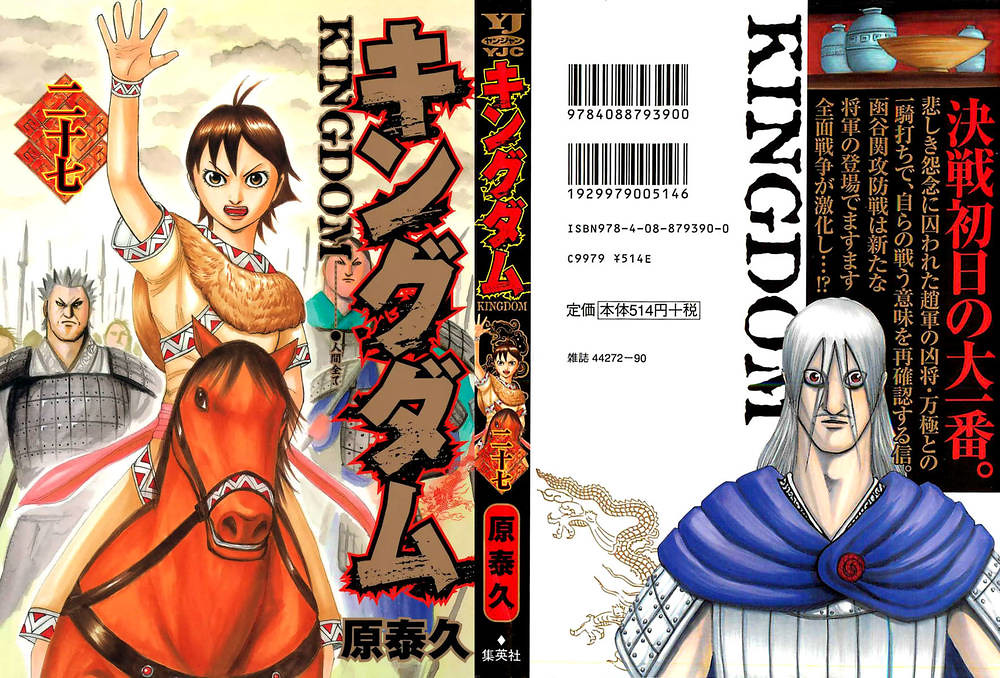The image appears to be a horizontally oriented, spread-out cover of an anime or manga titled "Kingdom," featuring both the front and back cover as well as the spine. On the left side of the cover, a young woman with short hair and dressed in a flowing outfit with a furry top is depicted riding a brown horse. Her right arm is raised with her hand open, fingers spread, as she seemingly leads an army, indicated by several figures holding spears behind her. The left side also includes Japanese characters along with the title "Kingdom" in English. The spine of the book, adorned with more Japanese characters, includes the acronym "YJC" at the top. On the right side of the cover, the back, there are multiple barcodes and an ISBN number. There is also an image of a man with long silver hair styled in two strands covering his face, wearing samurai armor and a blue robe draped over his shoulders. The overall design suggests a historical or samurai-era setting, rendered in a distinct anime or manga style.